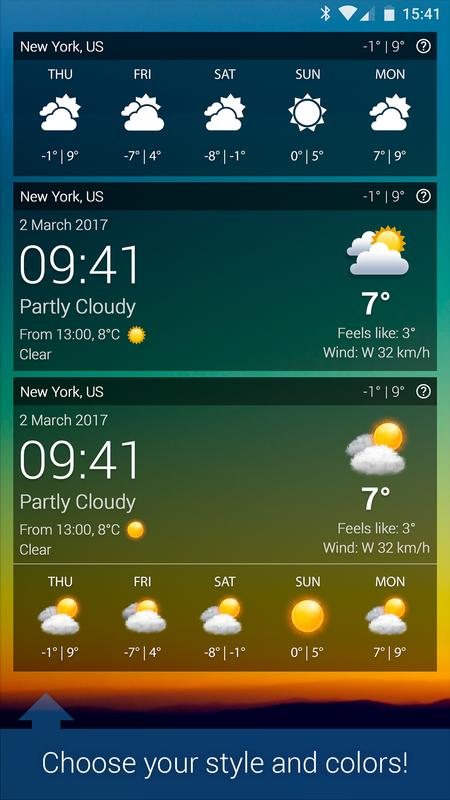This image appears to be a detailed mock-up or demonstration slide of a smartphone weather app interface, set against a background emulating an early sunrise. The gradient sky transitions from blue at the top through orange, ending in a hazy black horizon at the bottom, setting a calming tone.

Prominent in the foreground are three semi-transparent but slightly darkened panels, each showcasing different weather information. The panels and their mainly white icons and text contrast crisply against the dawn sky. At the top, the screen displays "New York, U.S." followed by a five-day weather forecast labeled Thursday through Monday. Each day is accompanied by weather icons and temperature readings.

In the central panel, today's weather for "New York, U.S." is depicted as "Partly Cloudy" with an image of the sun peeking through clouds, and a current temperature of 7 degrees. This panel reiterates that it is 9:41. 

The third panel consolidates the information from the first two panels, seamlessly integrating the detailed daily forecast with today's specifics.

Further below, a blue banner with white text invites users to "Choose your style and colors," featuring an upward-pointing arrow on the left, indicating customization options for the app. This implies that users can personalize the app's appearance, enhancing their interaction and experience.